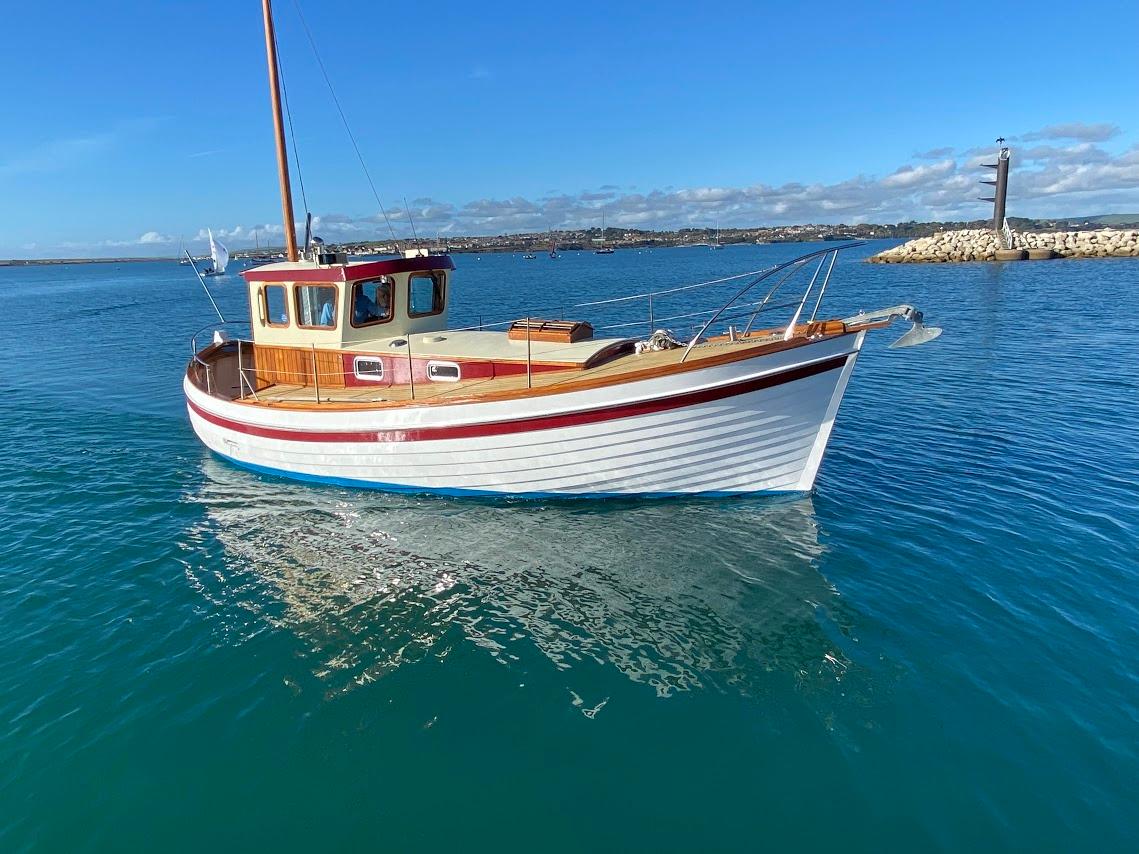The image depicts an older, small, personal wooden fishing boat with distinct features and an undeniable charm. The boat sits serenely on the water, which could be part of an ocean or bay, with visible land in the distance covered in structures reminiscent of a quaint, perhaps Mediterranean, area. The boat's hull is painted white with a striking red stripe running along its side, and the submerged portion is painted blue. Polished and stained wood enhances the top exterior, suggesting this is where people would walk. 

The boat's design includes a long, slightly downward-sloping front leading to a central cabin, which appears to have windows and offers some sheltered space beneath it. Notably, the deck features wooden elements and there are several poles, including a mast, hinting at its potential dual use as a motorized and sailing vessel. The reflection of this vessel on the calm blue water enhances its picturesque quality on a day marked by a blue sky dotted with some clouds. Additionally, the scene includes the presence of some distant boats, rocks to the right, and a light post, providing context and adding to the serene maritime setting.